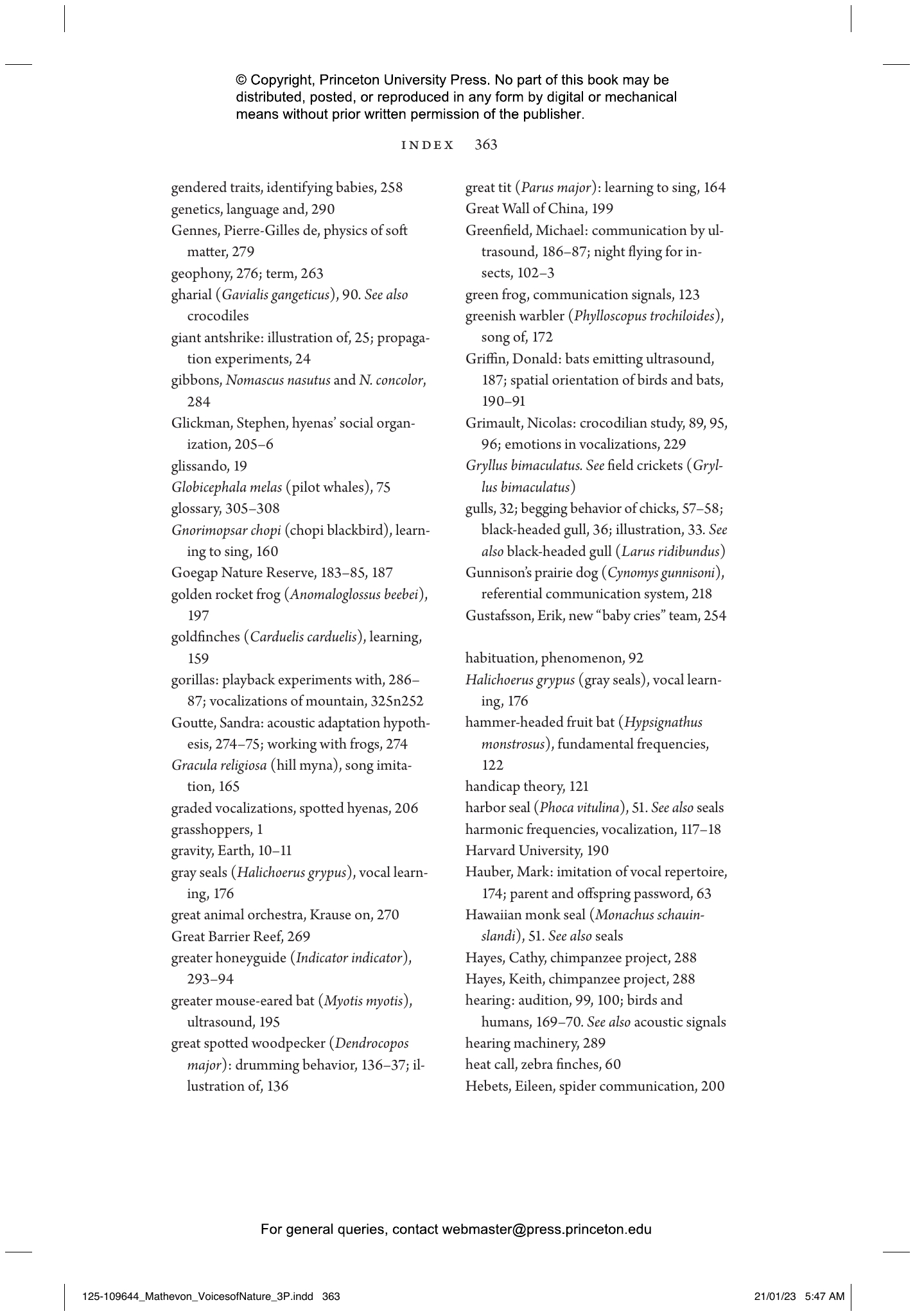The image depicts a page from the index section of a book published by Princeton University Press. The text is in black on a white background and is organized into two columns with hanging indents, typical of an index or reference book. At the top of the page, centered, are four lines of text in darker print that declare the page's copyright information, stating that no part of the book may be distributed, posted, or reproduced in any form by digital or mechanical means without prior permission from the publisher. The page also provides a contact email for general queries: webmaster at press.princeton.edu. Below this, the index entries are listed, showing terms followed by corresponding page numbers. Some entries include detailed phrases like "gendered traits identifying babies, 258" and "gravity earth, 10-11." The entries span across multiple lines with what appears to be around 15 entries per column.